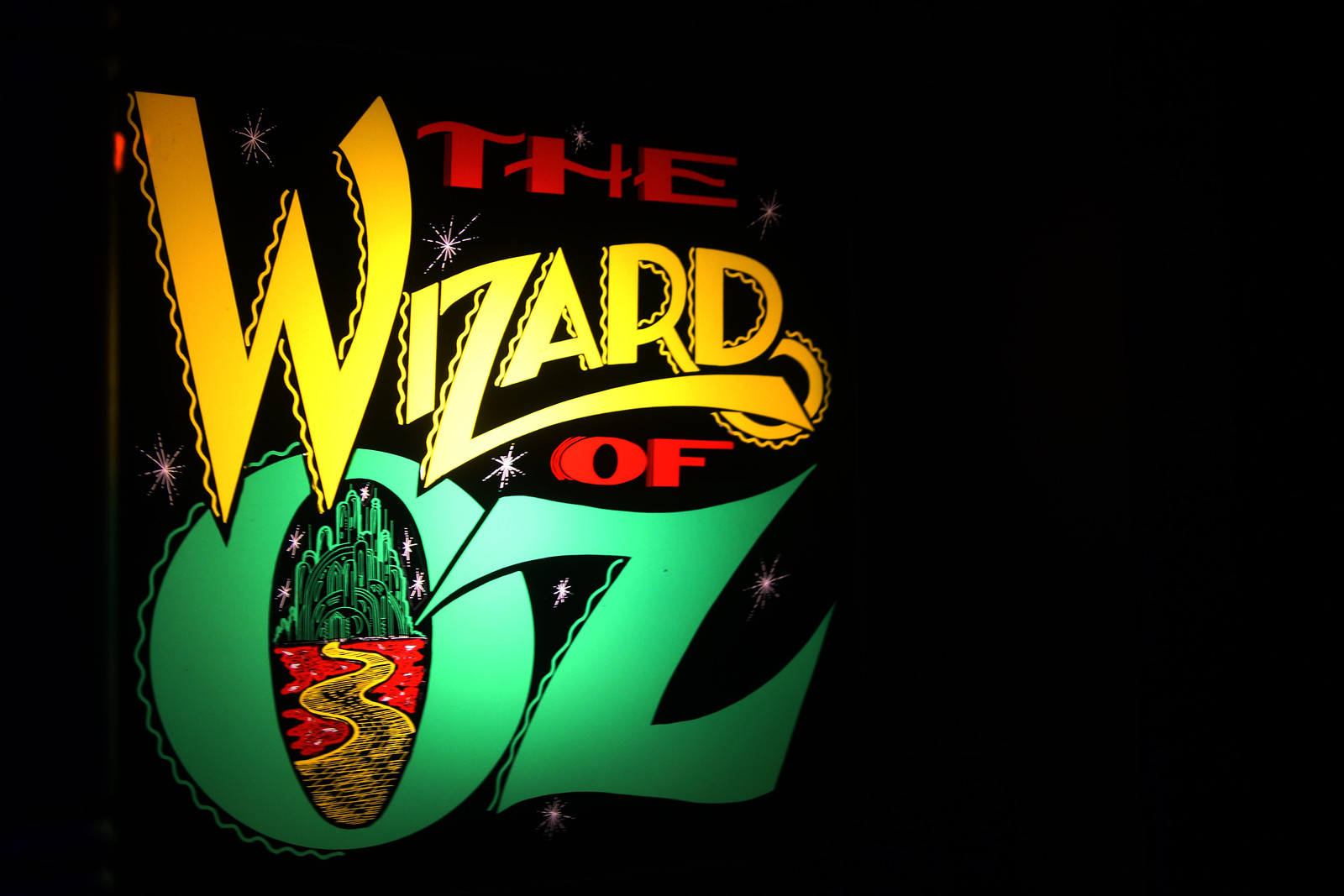The poster for "The Wizard of Oz" features a predominant black background, creating a dramatic and stark contrast that emphasizes the illuminated text and subtle details. Positioned mainly on the left side, the text "The Wizard of Oz" is displayed in large, bold letters. The word "The" is rendered in red, positioned at the top, followed by "Wizard" in yellow and immediately below it, "Of" reverts to red. Lastly, "Oz" is depicted in green and centrally placed. Enclosed within the letter "O" of "Oz," there's a detailed design depicting a golden path winding through a red and black landscape toward an iconic green castle, reminiscent of the Emerald City under a midnight sky. The entire sign appears to be lit by a strategic flash, highlighting primarily the text and the central illustration while leaving the rest of the image enveloped in darkness. This striking illumination gives the impression of a theatrical or club sign, possibly affixed to a building and designed to captivate attention at night. The large, exaggerated letters of "Wizard" and "Oz," adorned with stars and other decorative elements, dominate the composition, adding to the mystical allure of the poster.